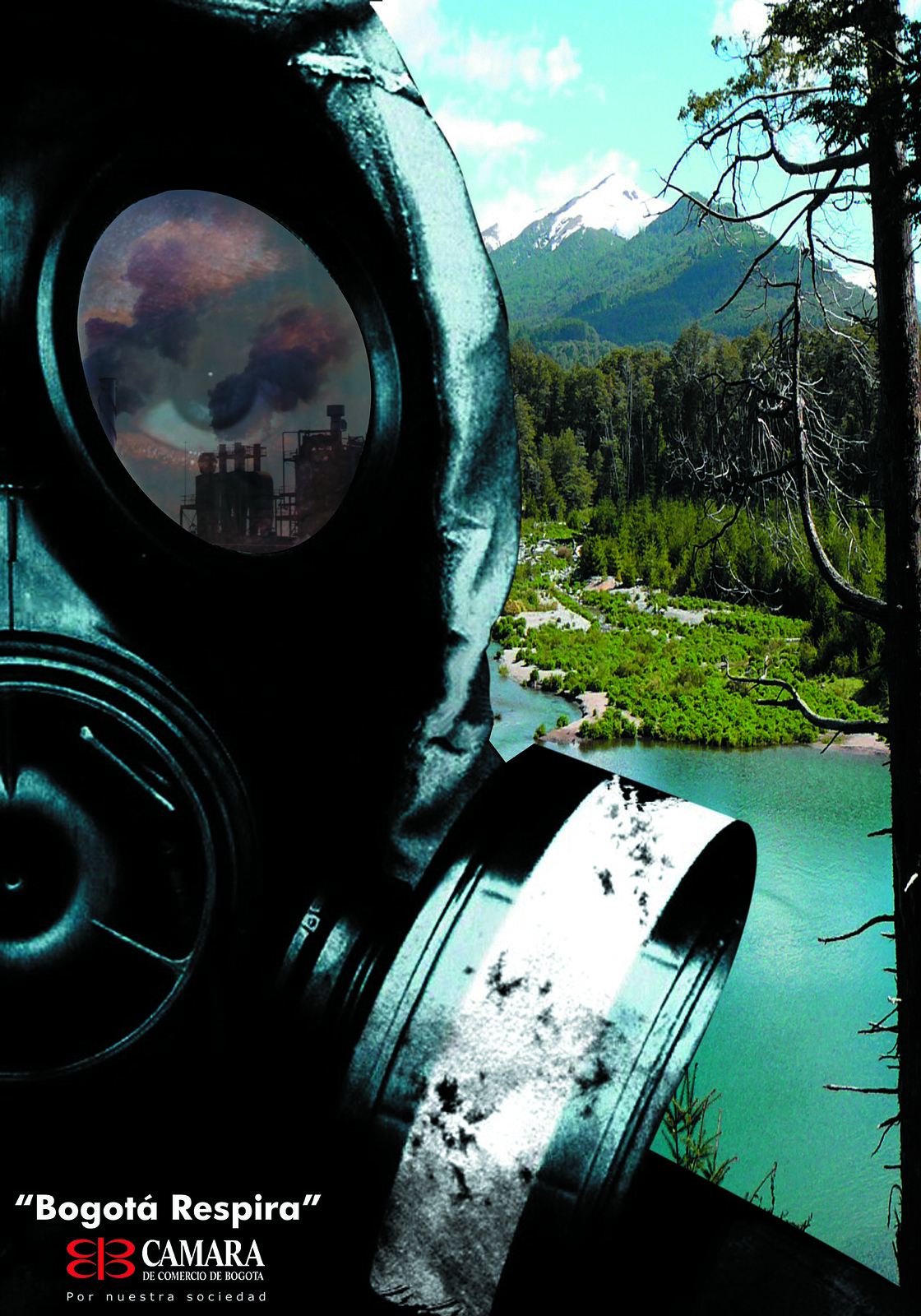The image is a close-up, computer-generated advertisement featuring a half-visible person wearing a black gas mask on the left side. The gas mask features large filters, and in the reflection of one of its lenses, you can see a factory with smoke billowing out. The scene behind the masked figure is a picturesque nature backdrop: a vibrant green landscape with a blue-green river meandering through it, tall evergreen trees, grassy areas, and a majestic, snow-capped mountain under a blue sky with scattered white clouds. The text "Bogota Respira, Camara" is displayed in the bottom left corner, along with a small, red, butterfly-like symbol and some tiny, hard-to-read lettering. The overall composition contrasts the stark, industrial reflection in the gas mask with the tranquil, natural scenery in the background.